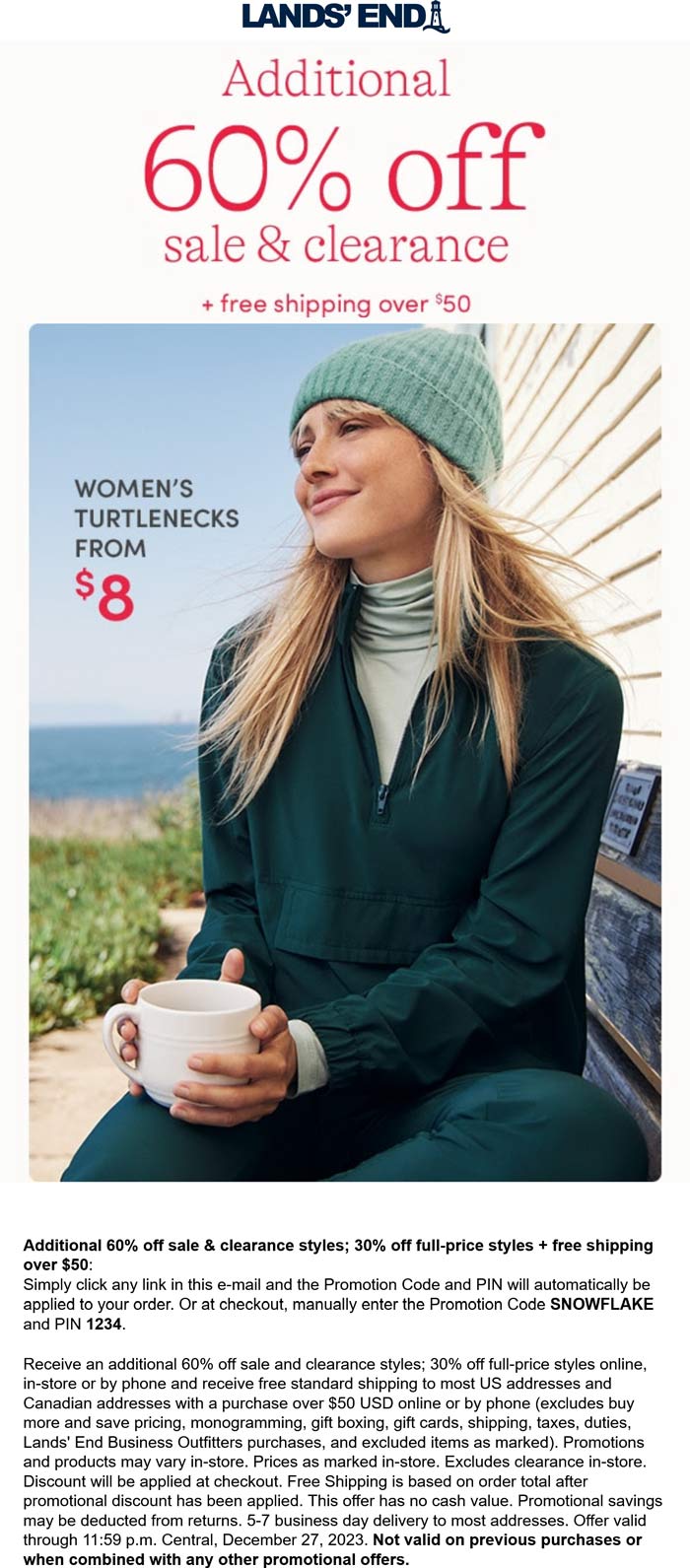This is a screenshot from a mobile phone showcasing an advertisement for Land's End, a clothing company. At the top of the ad, the Land's End logo is prominently displayed in bold, all-caps Futura font, featuring a small lighthouse icon at the end. 

Below the logo, the headline, shown in striking red text, announces a substantial promotion: "Additional 60% Off Sale and Clearance." Beneath this, smaller text highlights an added perk: "Plus Free Shipping Over $50."

Centrally positioned in the advertisement is a photograph of a woman dressed in various shades of green. She wears a turquoise cap, a light green turtleneck, and a dark green jacket paired with matching pants. The woman holds an empty cup, implying she might be enjoying a comforting beverage like coffee, tea, or hot chocolate. The setting suggests a chilly but clear day, as she sits on a bench outside a house. Behind her, there is an ice plant and a view of the ocean, with what appears to be an island visible in the distance under a blanket of clouds.

The bottom section of the ad is filled with an extensive amount of fine print, detailing the legal terms and conditions of the offer.